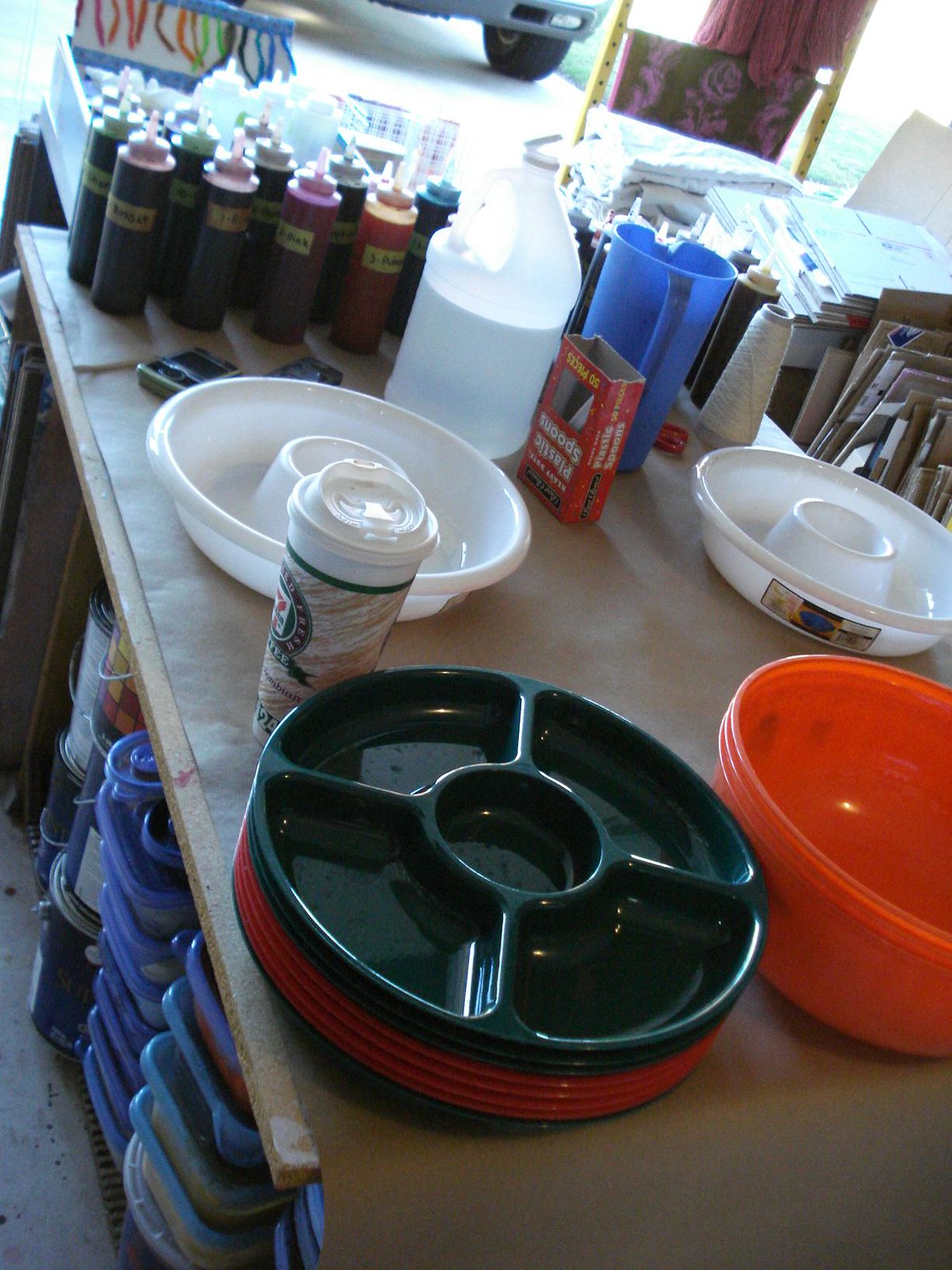The photograph captures a vibrant, well-organized workspace that appears to be dedicated to a creative craft, potentially jewelry-making or painting. 

In the foreground, there are several trays resembling plates, each featuring multiple slots radiating from a central circular groove, ideal for separating different beads or small materials used in necklace-making. The background is a burst of colors with an array of bottles, likely containing paint, given their varied hues. Among the assortment, a prominent blue pitcher for pouring water and a distinctive travel coffee cup branded with "7-Eleven" add character to the scene. A red bowl also rests on the table, standing out against the other items.

Beneath the table, several plastic bins with lids hold unseen contents, suggesting organized storage for materials or tools. On the tabletop, aside from the trays, there are white bowls and a spool of white string, further hinting at the intricacy and detail involved in the craft taking place here. The space emanates a sense of creativity and meticulous craftsmanship.